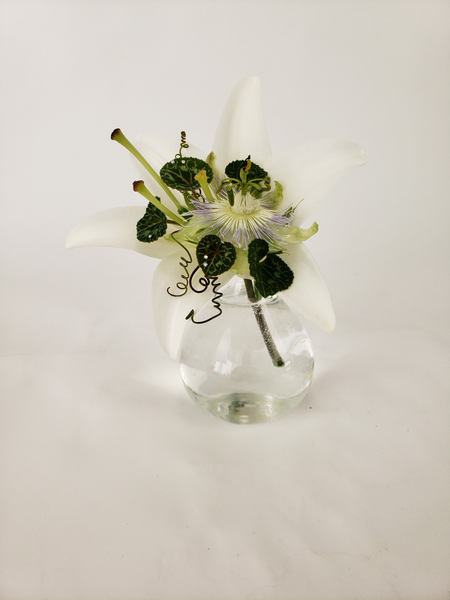This image showcases an artful presentation of a table setting, featuring a small, transparent glass vase that may be crystal. The glass vase, possibly oval-shaped with a darker gray base, is set against a pristine white background that could be either a tabletop or a tablecloth. The vase is filled with water, holding a single flower with white petals that have a purple tint at the ends. The flower’s green and curly stems extend into the water, and the vase is complemented by dark green leaves on the outside and lighter green leaves on the interior. There are additional decorative elements, like black petal-shaped pieces, including heart and circular forms, that add a sense of color and design to the composition. A faint white star in the background adds subtle texture, enhancing the overall visual appeal of this sophisticated tabletop piece.